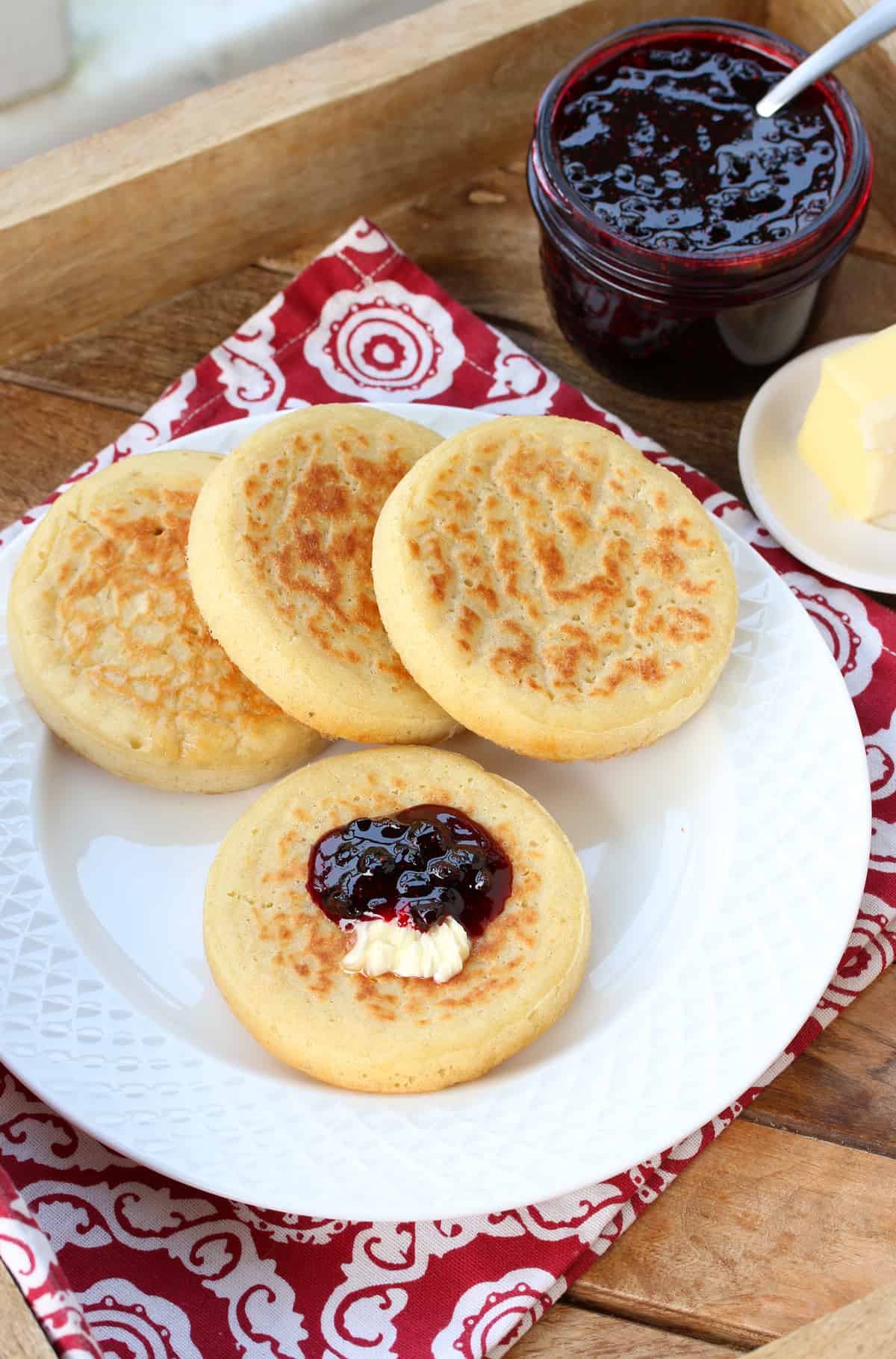This close-up photograph captures a cozy, country-style breakfast scene. Central to the image is a white plate placed on a red and white floral placemat, which itself rests on a brown wooden tray. The plate holds four light brown, circular English muffins with spots of darker browning where they've been toasted. One of the muffins is topped with a dollop of dark purple jam and a small piece of yellow butter. In the upper right corner outside the plate is a small white plate with a pat of yellow butter and a glass jar filled with dark purple jam, accompanied by a white or silver-handled spoon sticking out. The backdrop of the wooden tray complements the inviting rustic aesthetic.